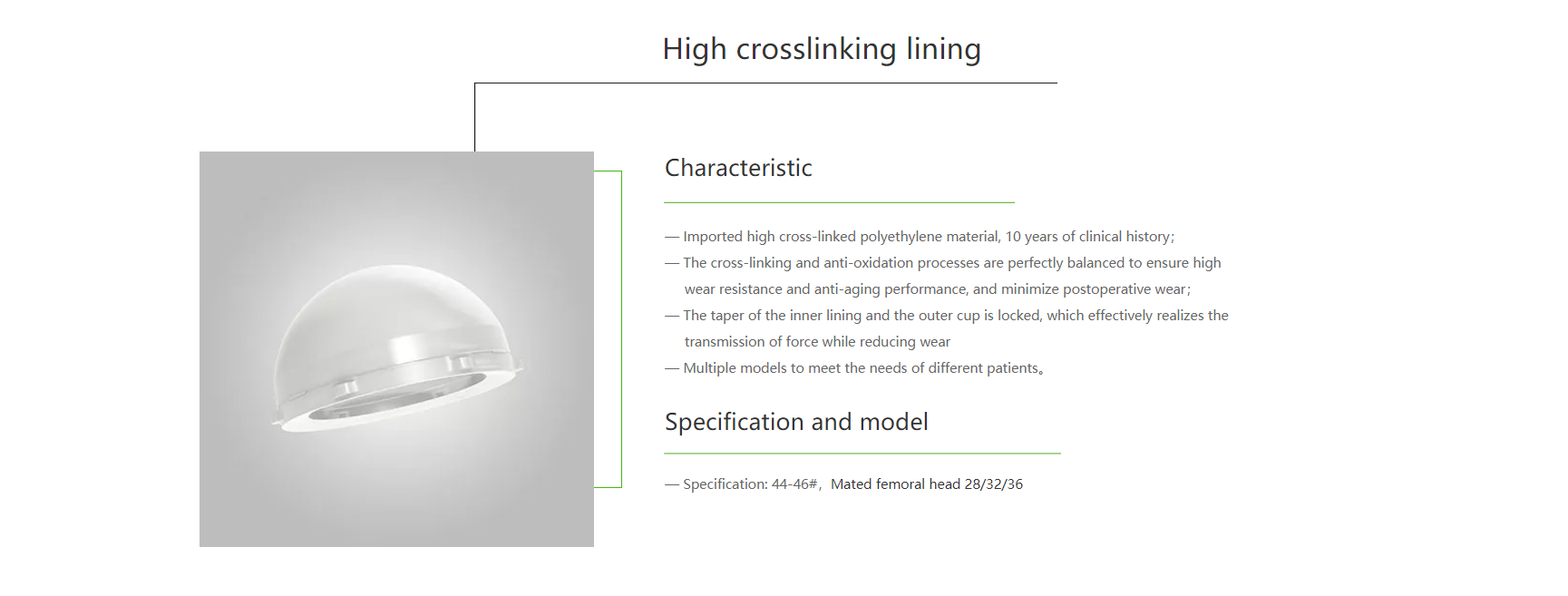The image showcases detailed information on high cross-linking polyethylene lining used in medical applications. On the left side, there is a gray shaded box displaying what appears to be the top portion of a hair dryer, with no additional context provided within this section. On the right, there's a comprehensive description that highlights the characteristics of the material used: imported high cross-linked polyethylene with a decade-long clinical history. The text emphasizes that the cross-linking and antioxidant processes are meticulously balanced to provide high wear resistance, anti-aging performance, and minimum post-operative wear. Additionally, the taper mechanism between the inner lining and outer cup ensures effective force transmission while minimizing wear. The product offers multiple models to accommodate the varying needs of different patients. 

The next section, labeled "Specification and Model," lists specific details: Description 44-46, with mated femoral head sizes of 28, 32, and 36. The information is clearly organized and easy to read, making it straightforward for potential users or medical professionals to understand.